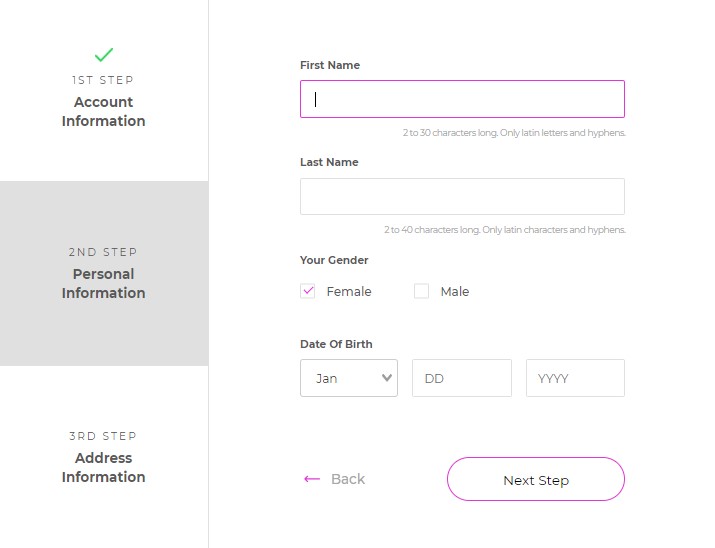Screenshot of an Account Setup Web Page

The screenshot captures a section of an account setup web page with a white background. The visible portion highlights the second step of a three-step registration process.

On the left side, the setup progress is displayed:
- The first step, labeled "Account Information," is marked with a green checkmark, indicating its completion.
- The current step, "Personal Information," is highlighted within a gray square.
- The upcoming step, "Address Information," is listed but not yet reached.

To the right, a section for entering personal information is shown:
- A labeled input field for "First Name."
- A labeled input field for "Last Name."
- A section for selecting "Gender," with radio buttons for "Female" and "Male"; "Female" is pre-selected.
- A field for "Date of Birth," featuring a drop-down menu for the month and text fields for the day and year.

At the bottom right of the form, there is a rectangular button with rounded edges labeled "Next Step."